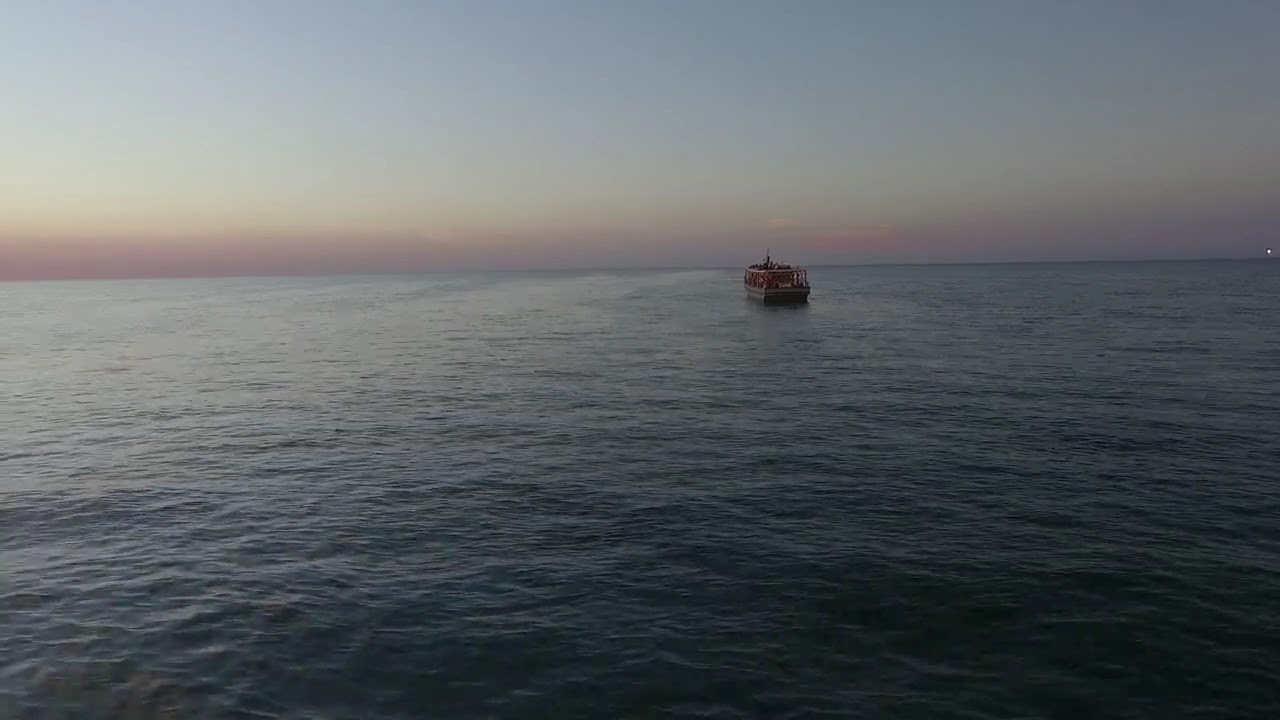In the photograph, an expanse of the open ocean with calm blue waters stretches into the distance, meeting the horizon at the top third of the image. The sky is devoid of clouds and exhibits a gradient of colors, transitioning from a deep purple near the horizon to a lighter blue and eventually a whitish hue, indicative of either a sunset or dawn setting. Central to the image is a distant boat, appearing to be a barge, ferry, or tugboat. This vessel features a black base, reddish vertical bars or railings, and a white roof. These details suggest it's navigating away from the camera. Gentle waves ripple across the ocean's surface, emphasizing the tranquil nature of the scene. Near the horizon, just to the right, a faint light can be spotted, possibly emanating from another boat or a distant landmass. The overall serenity is accentuated by the clear, open sky and the soft, pinkish tint along the horizon.